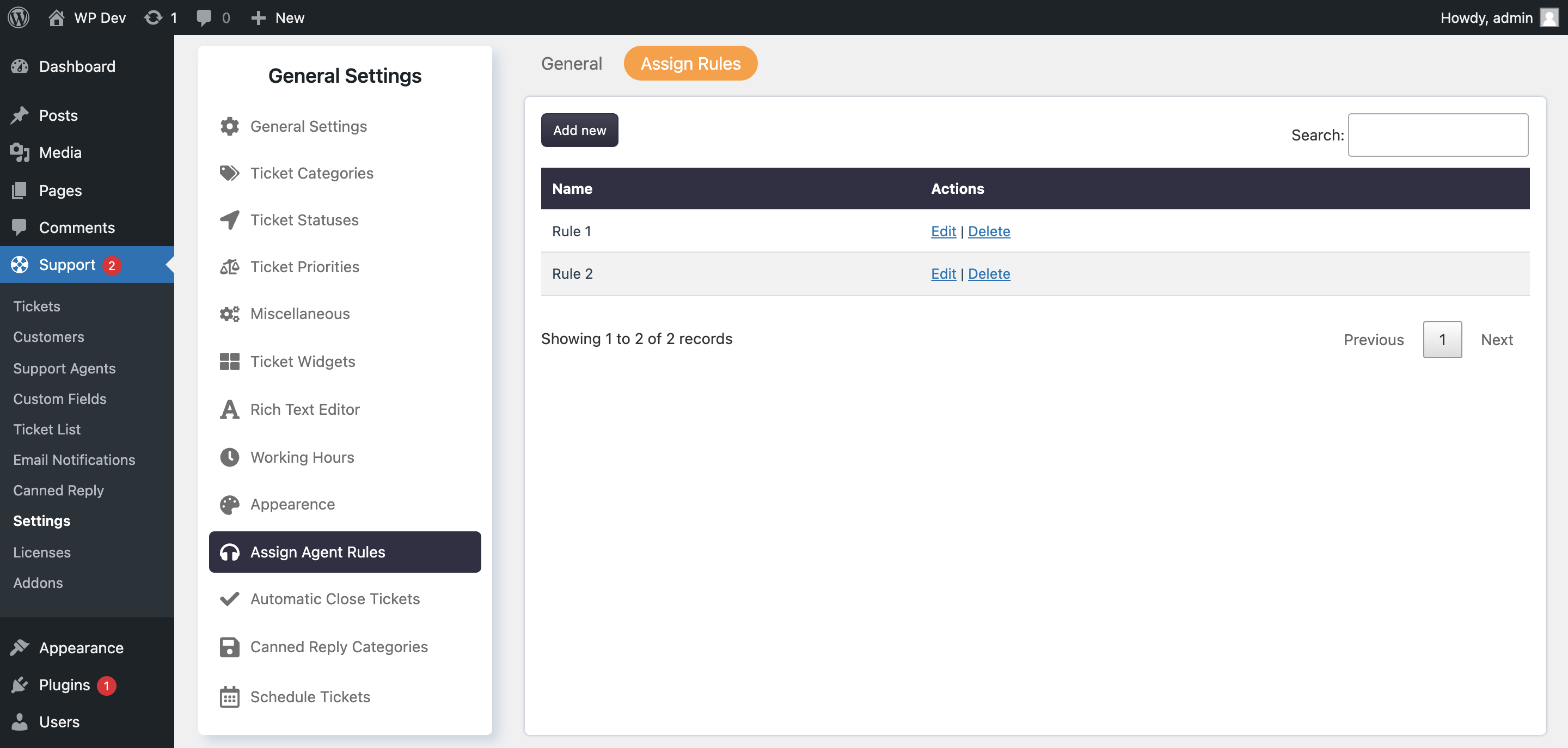**Detailed Caption:**

The image showcases a settings interface, likely from a computer or website dashboard. The left-hand sidebar features an extensive menu with several options listed vertically. The options include:

1. Dashboard
2. Posts
3. Media
4. Pages
5. Comments
6. Support (highlighted in blue with a red notification circle displaying the number '2')

Under the 'Support' section, the following sub-options appear:

- Tickets
- Customers
- Support Agents
- Custom Fields
- Ticket Lists
- Email Notifications
- Canned Reply
- Settings (highlighted in bold white)
- License
- Add-ons

Further below, additional menu items include:

- Appearance
- Plugins (with a notification circle displaying the number '1')
- Users

A box adjacent to the sidebar, labeled 'General Settings,' lists subcategories related to settings:

- General Settings
- Ticket Categories
- Ticket Statuses
- Ticket Priorities
- Miscellaneous
- Ticket Widgets
- Rich Text Editor
- Working Hours
- Appearance
- Assign Agent Rules (outlined with a black box, indicating it is the selected subcategory)
- Automatic Closed Tickets
- Canned Reply Categories
- Schedule Tickets

The main content area of the interface is divided into sections. The top section, labeled 'General,' has a highlighted 'Assign Rules' option in orange. Below, there is a button labeled 'Add New' followed by columns for 'Name' and 'Actions.'

The 'Name' column lists 'Rule One' and 'Rule Two.' The 'Actions' column provides options to either 'Edit' or 'Delete' the listed rules. At the bottom, the interface indicates that it is displaying records 1 to 2 out of a total of 2 records, confirming that there is only one page of data.